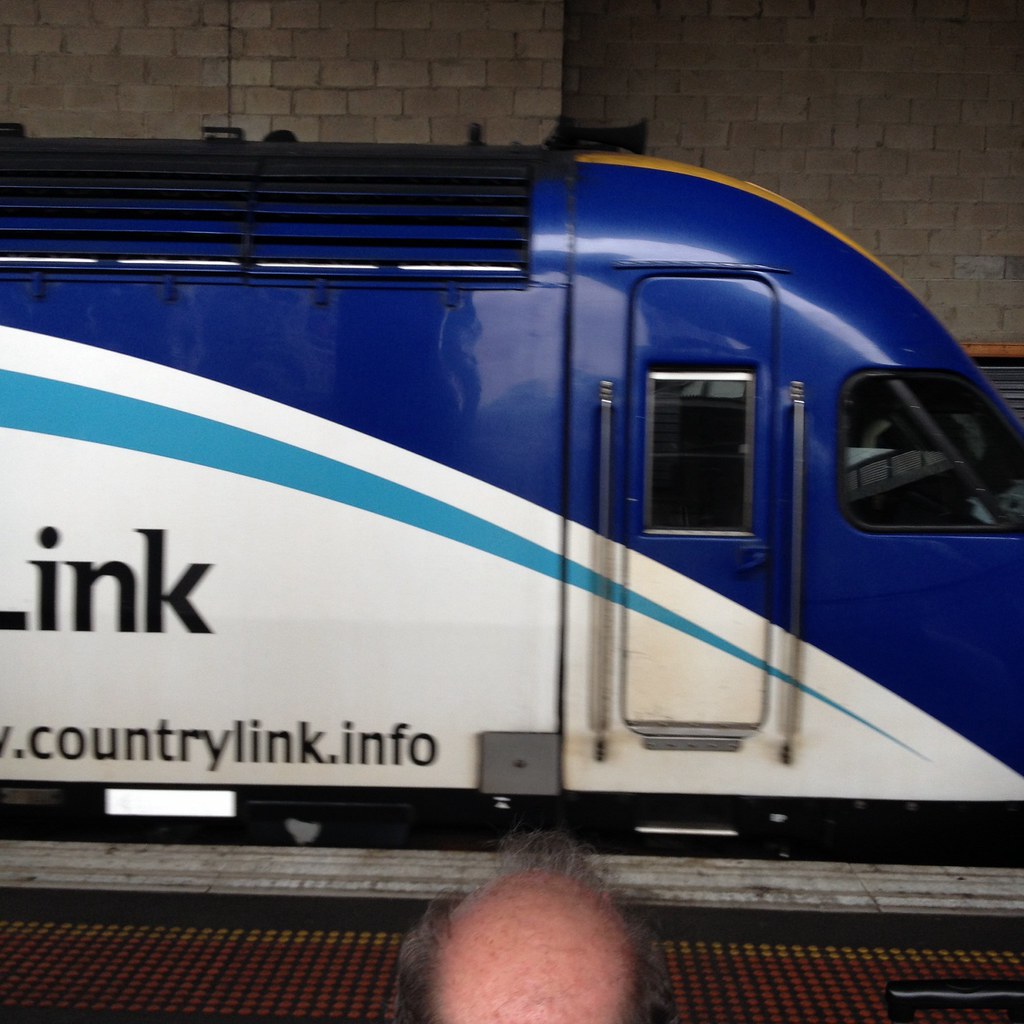The image depicts a close-up view of the front of a modern train stationed at what appears to be an underground subway platform. The train is primarily blue and white, with a dark blue top that slopes down to a pointed front. Just visible on the train's front are the partial letters "L" and "INK," followed by "countrylink.info" in black letters against a white background. The train's windshield and the door leading to the driver's compartment are noticeable, though partly obscured by reflections. Directly in front of the train is part of the platform, which features a patterned area with red dots and yellow markings for secure foot traffic. In the foreground, the balding head of an older man with fluffed-up gray hair is centered at the bottom of the frame. The man's presence suggests he might be waiting to board the train. Venting is visible on the top left of the train, characterized by dark vent openings and gaps between the metal slats. The overall setting includes a gray stone wall in the background, adding to the underground ambiance.